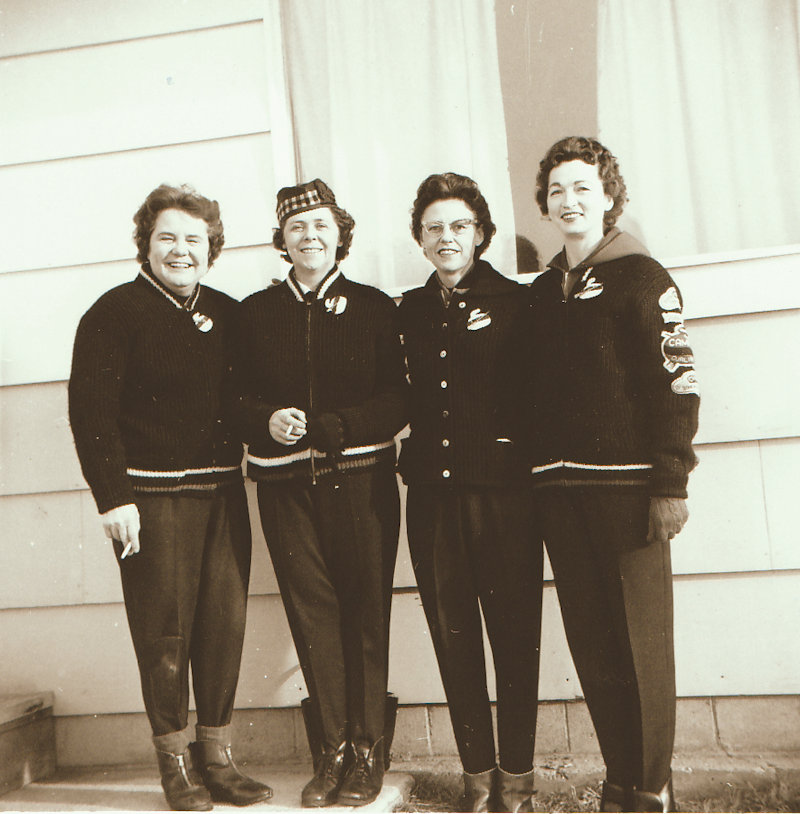This vintage, sepia-toned photograph captures four smiling women standing in front of an off-white house with large windows adorned with white curtains. All four women are clad in uniform-like outfits consisting of black jackets with white trim around the collar and bottom, black pants, and brown shoes, indicating a sense of camaraderie or shared activity. Their short brown hair frames their faces, giving a snapshot of mid-20th-century style. 

The first two women on the left are holding cigarettes, adding an air of casual leisure. The second woman wears a black hat with a checkered band, and she stands on a patch of gray concrete alongside the first woman. She is also notably wearing gray gloves, perhaps indicating chilly weather. The woman next to her, wearing distinct cat-eye glasses, and the one on the far right, who is wearing a jacket with a hood, are positioned on a grassy part of the scene. The jackets appear to be warmly knit, suggesting a cold climate, potentially hinting at the setting being somewhere like Scotland. The overall attire and accessories, such as the cat-eye glasses and the checkered hat, suggest that the photograph dates back to the 1950s.